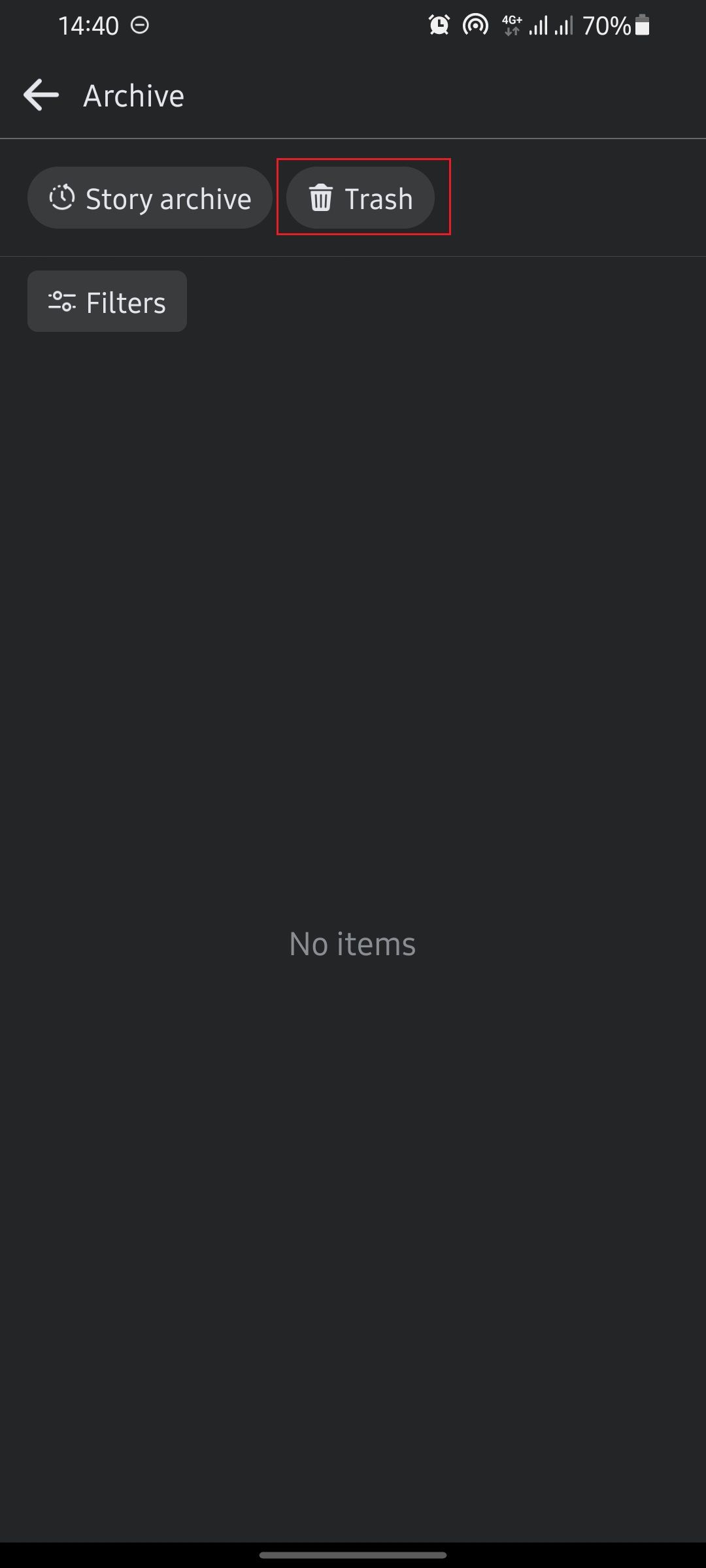The image appears to be a screenshot from a phone, given the visible status bar at the top indicating it is 14:40. The status bar also shows various icons, including a white circle with a line through it, a circular icon with concentric lines, a strong 4G signal indicator, and a battery icon at 70% charge.

The main content of the screenshot displays a section labeled "Archive." Directly below this, there is a back arrow icon in white, pointing to the left, followed by a gray line. Below this line, the text "Story Archive" is prominently shown in white, flanked by a white clock icon. To the right of this, there is a white trash can icon with the word "Trash" in white letters inside a red square.

Further down, there is an option for "Filters," denoted by two lines and two bars in white, accompanied by the word "Filters" in white text. The rest of the screen is largely empty except for the phrase "No items" displayed in gray letters. The entire screen features a monochromatic color scheme consisting of black, white, and gray tones.